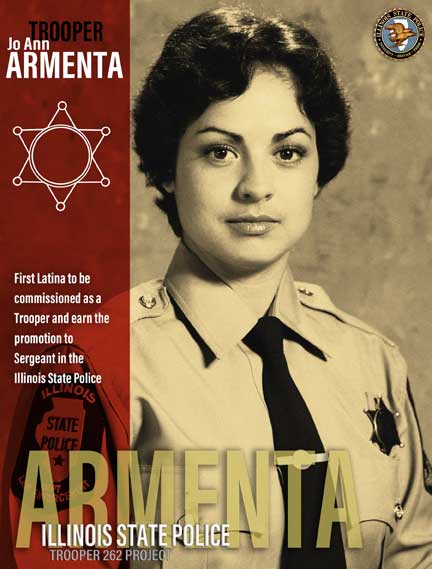This is a black and white headshot photograph of Illinois State Police Trooper Joanne Armenta, featured as part of the Illinois State Police Trooper 262 Project. She is the first Latina to be commissioned as a trooper and earn the promotion to sergeant in the Illinois State Police. The image shows her in a sheriff's uniform with a button-down shirt, a black tie, and a badge on her left chest. She has short black hair and is looking directly into the camera. The background of the magazine cover is split, with the left 40% in red and the right 60% in a tannish color. The text over the red background includes "Trooper" in black, followed by "Joanne" and "Armenta" in white. Below are her achievements, also in white text, highlighting her historic milestone within the force. The upper right corner of the image features the Illinois State Police seal.